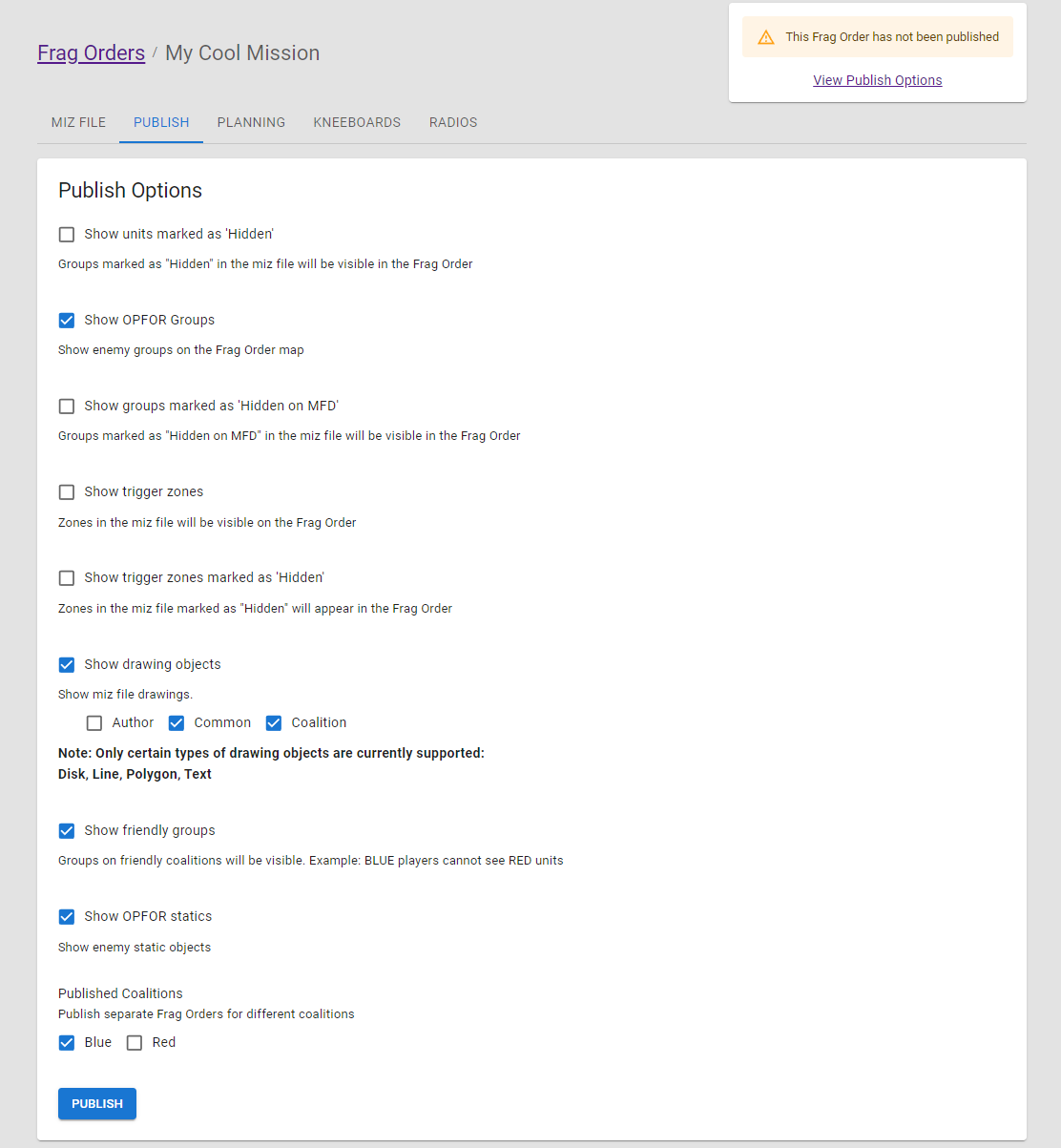In this detailed caption, we're describing a screenshot of a web page designed for file publishing. The outer edges of the image - on the left, right, and top - feature a gray background, while the majority of the image has a white background. 

At the top right corner of the image, there is a notification that reads, "This flag order has not been published," followed by a clickable link in bluish-purple text that says, "View Publish Options."

On the left side of the image, a sidebar includes a menu with a highlighted section in purple labeled "Frag Orders." Beneath this, there are other categories like "My Cool Mission," "Mid File," "Miss File," "Publish," "Planning," "Kneeboards," and "Radios," with "Publish" currently selected.

In the main section of the page, under the heading "Publish Options," there are nine different publishing options. Some of these options are selected, indicated by blue squares with white checkmarks. Others remain unselected, shown as white squares without checkmarks.